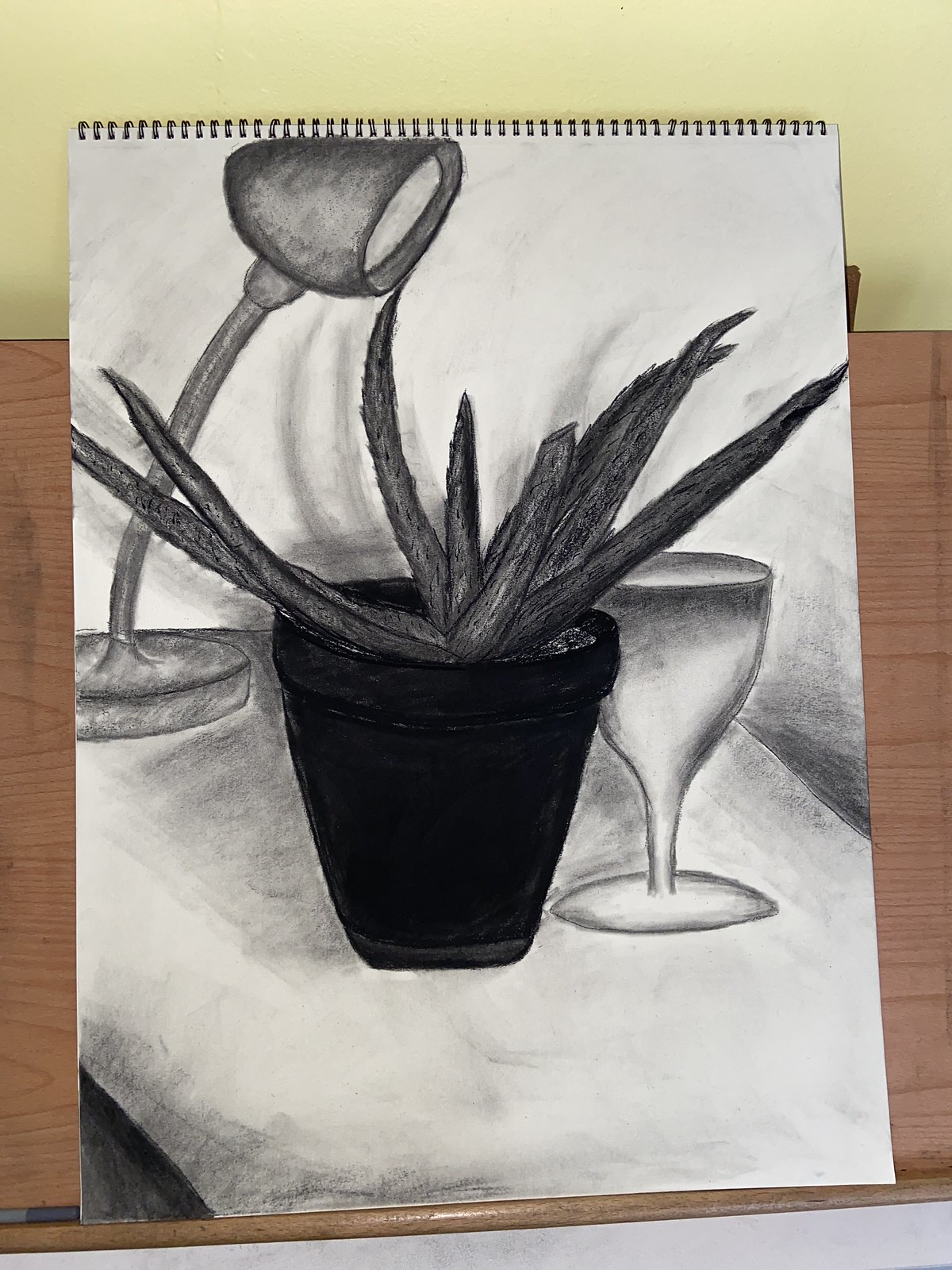This detailed sketch depicts a still life scene featuring a potted plant, a wine glass, and an overhead lamp, all arranged on a table. The composition is notable for its dramatic shading and use of grayscale tones. Dominating the center of the image is a pot, heavily shaded in black, creating a stark focal point. Emerging from the pot are elongated leaves, markedly dark, resembling blades of grass. To the right of the pot stands a wine glass, shaded with a gradient from dark gray at the top to a lighter gray at the bottom. On the left side of the composition, an overhead lamp, also shaded in gray, adds balance to the scene. The table beneath these objects is lightly shaded in gray, with darker shading behind the pot adding depth to the sketch. Above, the black rings of a notebook are visible, indicating the drawing's setting within a sketchbook. The broader surroundings include a brown table surface and a tan-colored wall, framing the still life contextually.